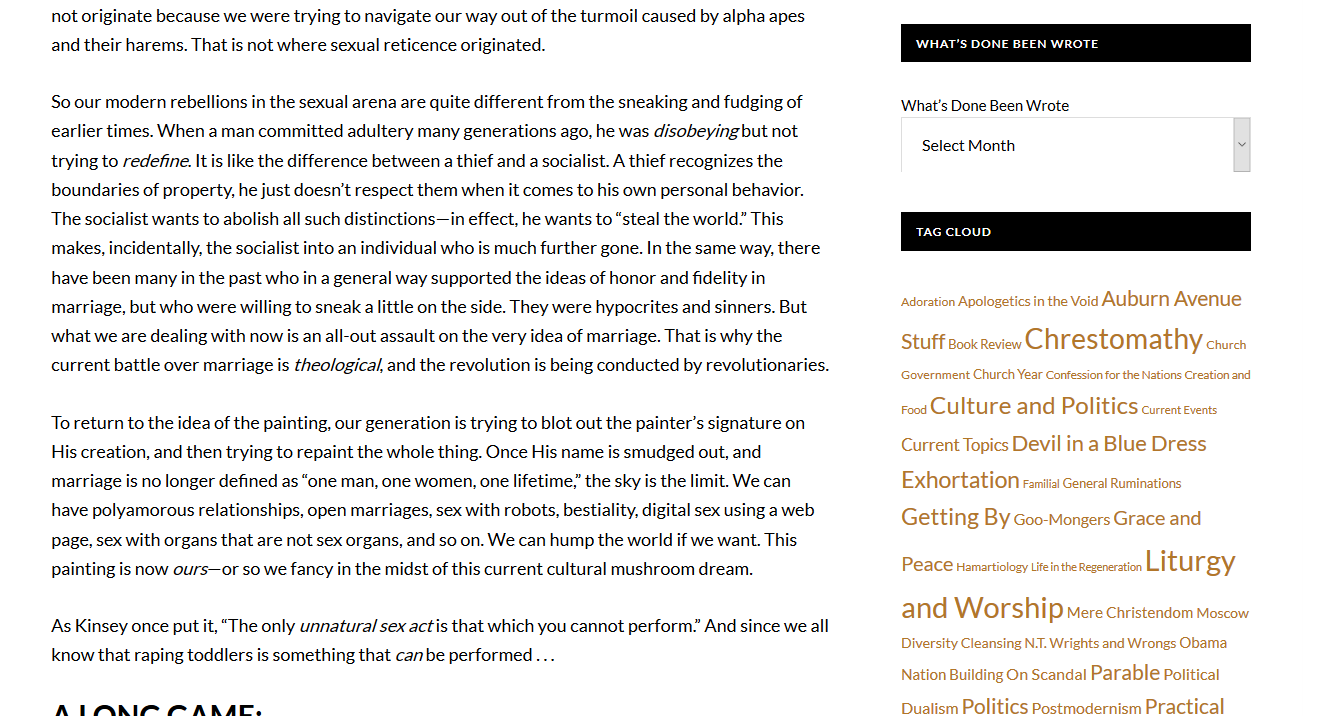The image depicts a webpage, likely not the homepage but an inner page. The text begins abruptly with a discussion on the origins of sexual reticence, debunking the notion that it began as a response to alpha apes and their harems. This introduction spans two paragraphs. 

At the end of these paragraphs, there is a bolded word in all caps, partially obscured, rendering it unreadable. To the right, a vertical black bar displays text. The primary phrase, written in various colors including pink, yellow, and blue, reads, "What’s done been wrote." Below this, you can select a month from a drop-down menu, labeled with something that includes the word "cloud" in another black bar at the bottom. 

A subsequent paragraph exhibits a striking visual style, featuring words in different sizes—ranging from small to very large—with alternating sizes throughout, all rendered in gold.